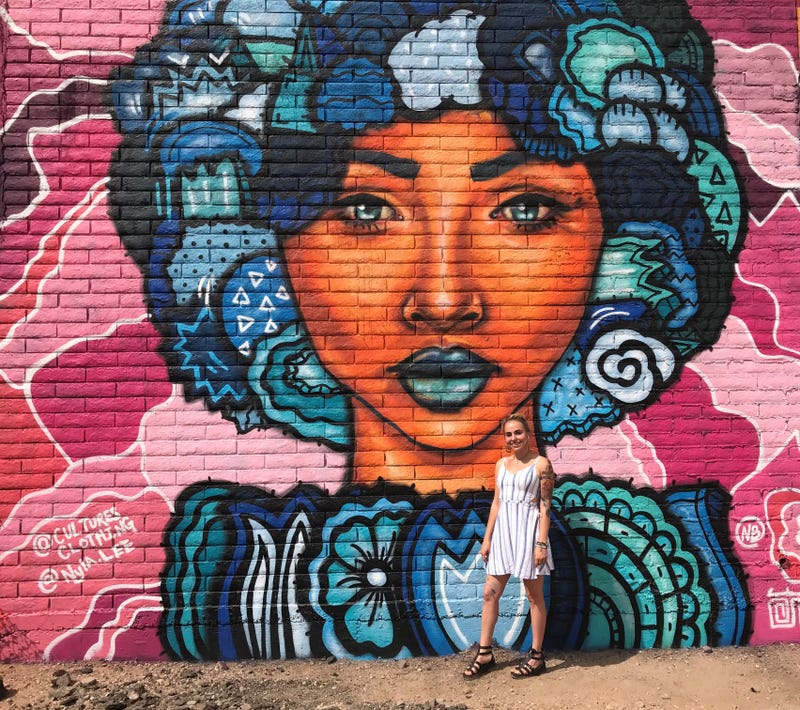This photo, taken outside during the day, captures a young lady standing in front of a vibrant, graffiti-adorned brick wall. She is clad in a white and blue striped sundress and sandals, with her hair pulled up and tattoos visible on her arm. The mural behind her is a stunning depiction of a black woman with intricate blue hair, composed of floral-like designs in varying shades of blue. The woman in the mural has piercing blue eyes, blue lips, and a blue and green flower necklace. The background of the mural features pink camouflage patterns. The left side of the wall displays the text "@culturesclothing" and "@nia.lee." The overall ambiance suggests it's a warm day, likely fitting for a casual stroll through the city.